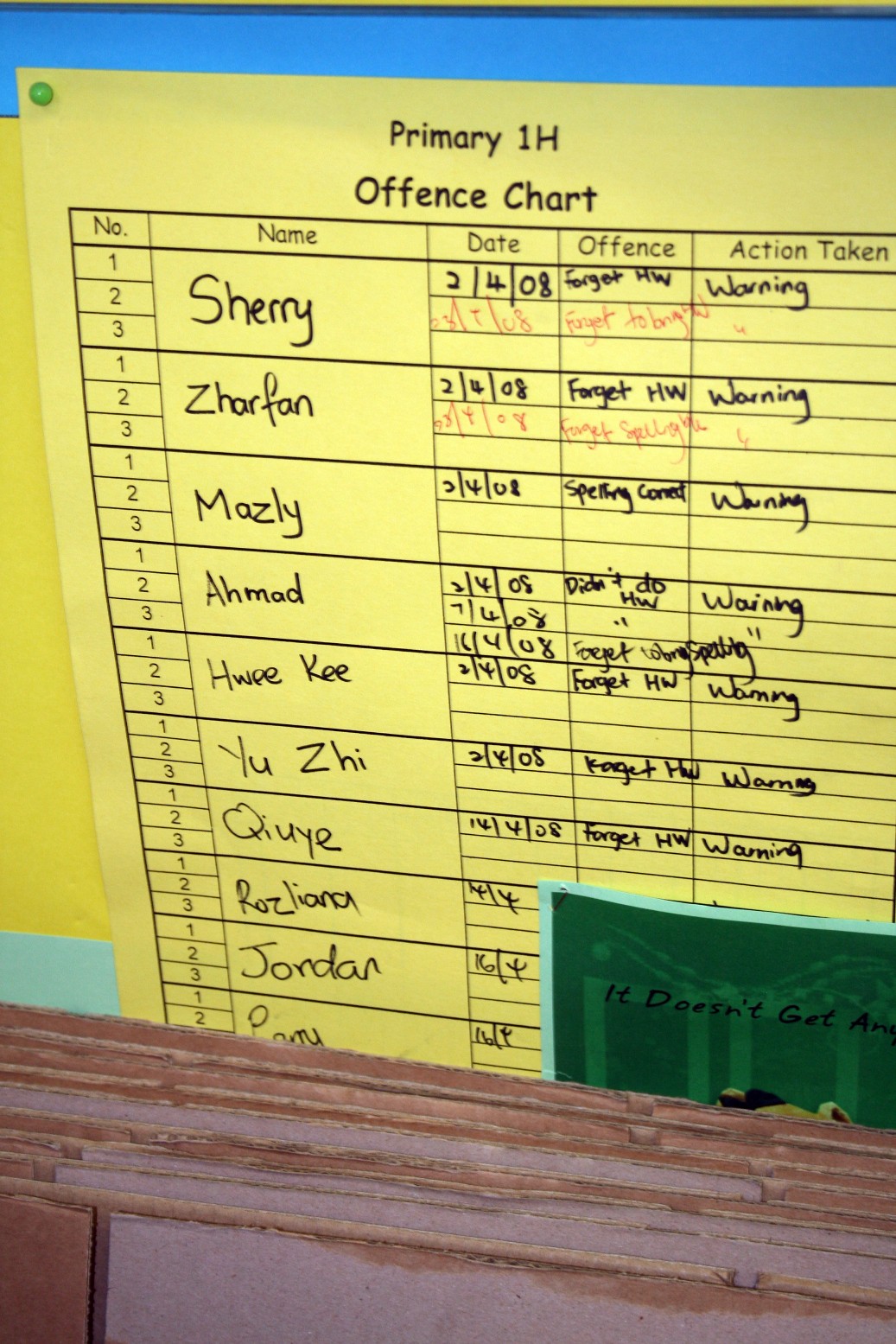The image features a yellow piece of paper thumbtacked to what appears to be a wall. At the top of the paper, in black writing, it reads "Primary 1-H Offense Chart." The chart is organized into five columns labeled: Number, Name, Date, Offense, and Action Taken. There are a total of ten individuals listed on the chart, including Sherry, Zarfan, Masley, Ahmad, Hui Kee, Yuzi, Kuyi, Rosliona, and Jordan. 

Each person has at least one date associated with their name, with Sherry and Zarfan having two dates, and Ahmad having three. The dates primarily read 2-4-08, indicating the day they were warned. The 'Offense' column details the specific infractions, while the 'Action Taken' column consistently lists "Warning" next to each individual. 

The chart is pinned above another green piece of paper, partially visible and cut off at the bottom, bearing the text "it doesn’t get A.N." The entire setup appears to be on a wooden surface, possibly a desk.